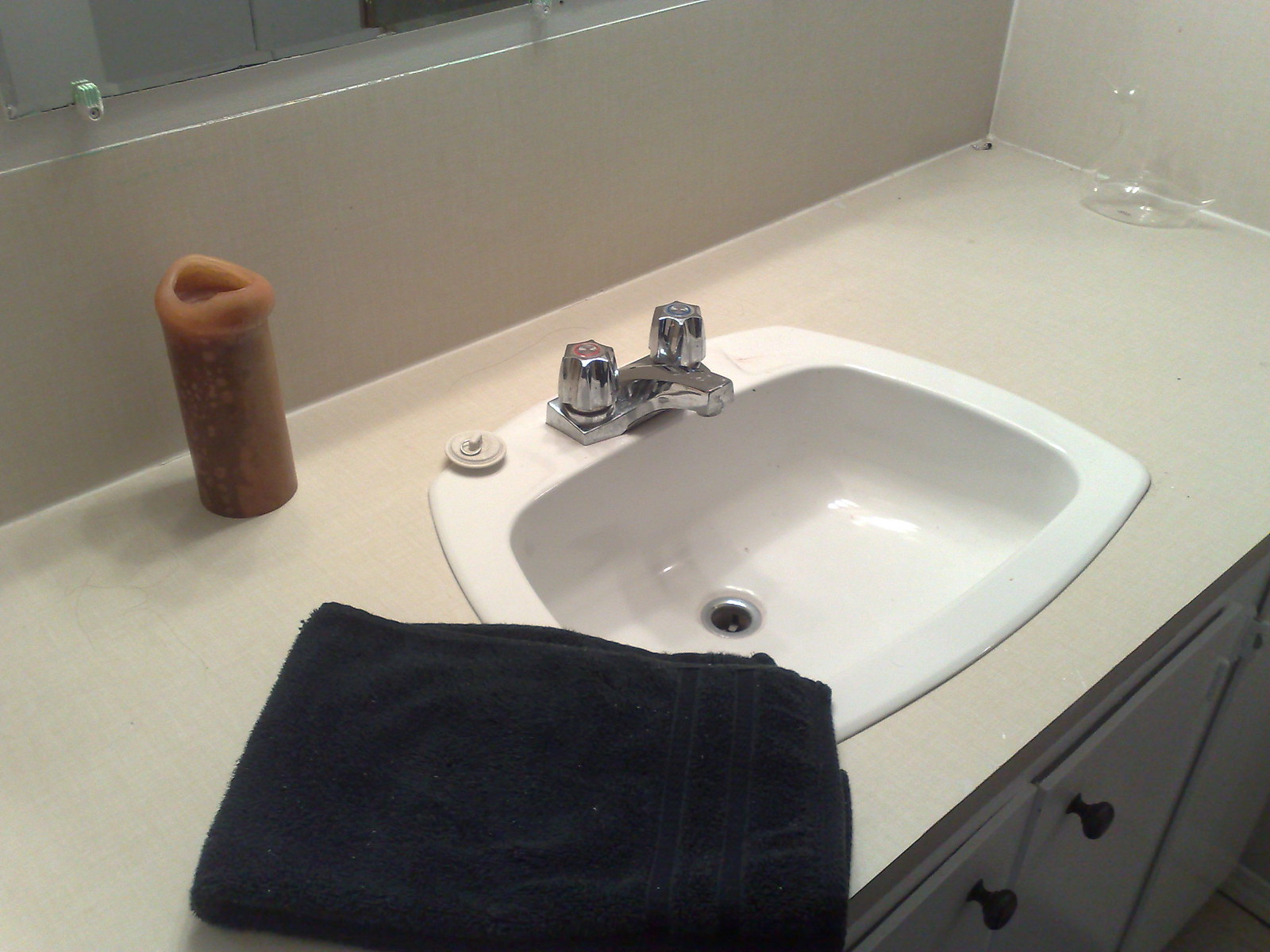The image captures a well-organized bathroom sink area. The off-white countertop features a neatly folded dark-colored towel spread partially over the sink and countertop. At the back of the sink, a tall butterscotch-colored candle adds a warm touch to the space. The bottom section of a wall-mounted mirror is visible, reflecting part of the setup. The white porcelain sink, with its modern square design, stands out prominently. Positioned on top of the sink is the sink stopper, and the hot and cold water valves are clearly visible along with two sleek handles for water control. Below the sink, the image shows two front-facing cabinet doors, offering storage space. To the far left of the image, a glass jar or vase is placed next to the sink, adding an additional decorative element to the scene.